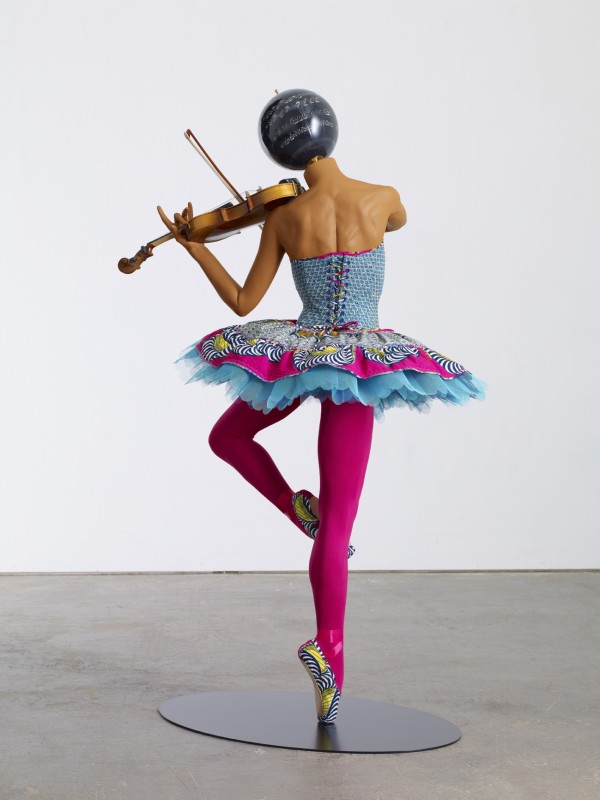The image features a detailed sculpture of a headless ballerina, posed elegantly on a single black circular base. The background is a pure, solid white, contrasted by the cement-gray surface on which the base rests. The ballerina is captured mid-pose, standing en pointe on her right toe, with her left leg bent and crossed in front of her right knee. She wears striking ballet shoes adorned with black and white stripes, accented by yellow decorations. Her legs are covered in bright pink tights.

The ballerina's outfit is vibrant—a blue tutu, which includes a blue underskirt layered with a pink overskirt, adorned with various blue and black circles. Despite the mannequin-like appearance of her form, an absence of a human head is replaced with a smooth, gray, head-sized marble, perhaps etched with barely discernible markings. In her right hand, obstructed by her torso, she delicately holds a golden violin, while her left arm extends gracefully, guiding the bow across the strings. The overall composition, blending whimsical attire with a poised, expressive stance, creates a captivating artistic piece.